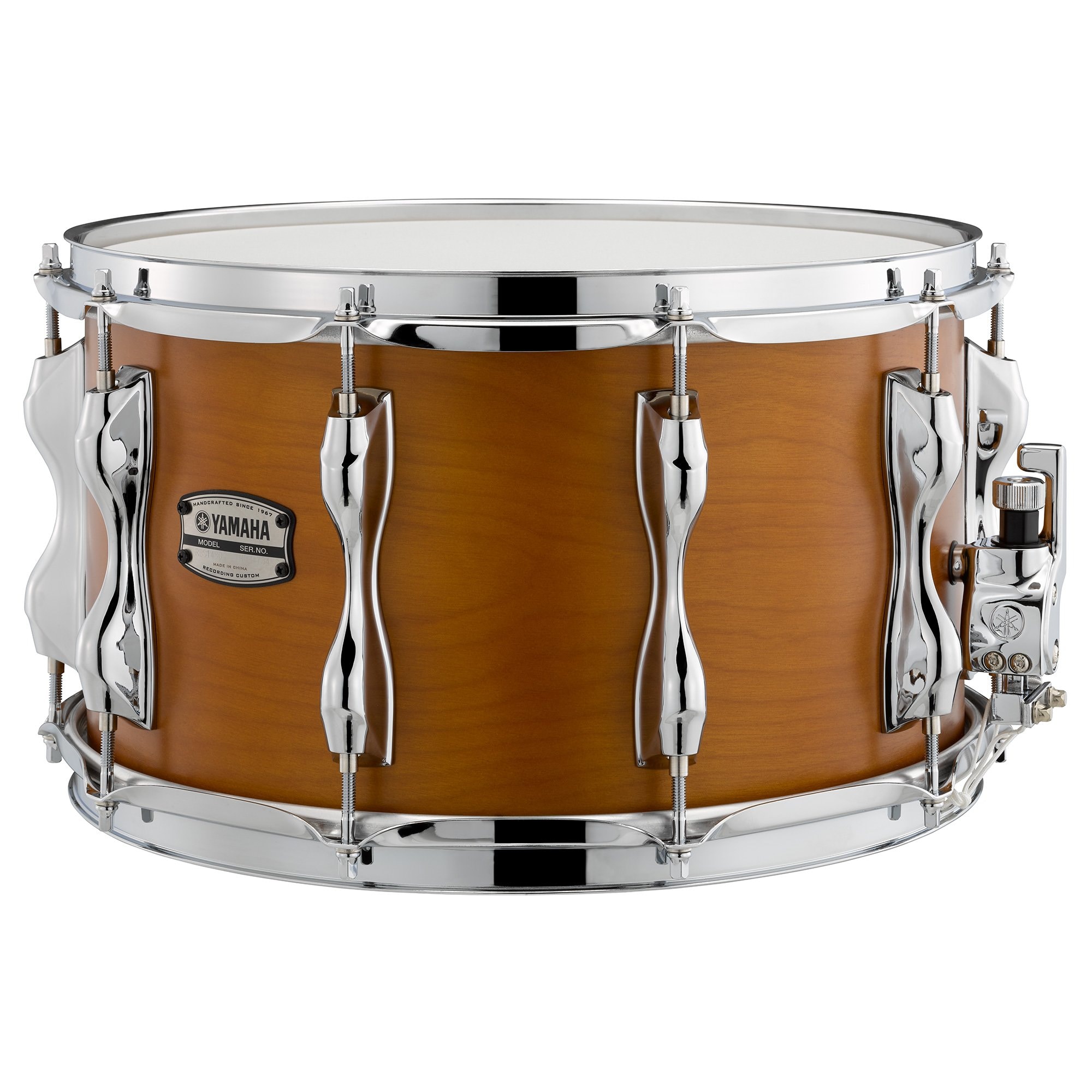This detailed photograph showcases a Yamaha snare drum with a medium-sized, cylindrical body featuring a light brown wood grain pattern. The drum is adorned with a stainless steel trim and multiple evenly spaced, long silver metal pieces that secure the white drumhead, or skin, to the frame. A prominent, square, silver and black plaque reading "Yamaha" is positioned on the left-hand side of the drum. The drum appears to be new and well-maintained, set against a plain white background that accentuates its polished components. The stainless steel adjusters and tuning mechanisms are visible, along with several screws and reflective details near the bottom, giving the drum a refined and high-quality appearance.